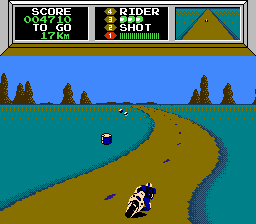This detailed screenshot from an 8-bit retro motorcycle racing game depicts a motorcyclist navigating a curvy, orange-brown dirt road bordered by dark blue dashed lines. The road is flanked by grass that is highlighted in various shades of blue. Scattered along the road are cylindrical objects featuring dark blue and white colors, with more appearing in the distance. In the background, silhouetted brown and black trees contrast against a cyan blue sky. The motorcyclist is wearing a blue shirt with black details and a white helmet adorned with a blue stripe. The top portion of the screen displays a gray rectangle with white text: "SCORE 004710 TOGO 117KM." Adjacent is another rectangle that reads "4RIDER 3" with three circles containing smaller white circles, and "2SHOT 1" accompanied by a green hash-marked bar where the number "1" is in red. The far right features a small map illustration showing the road and a smaller depiction of the motorcyclist.